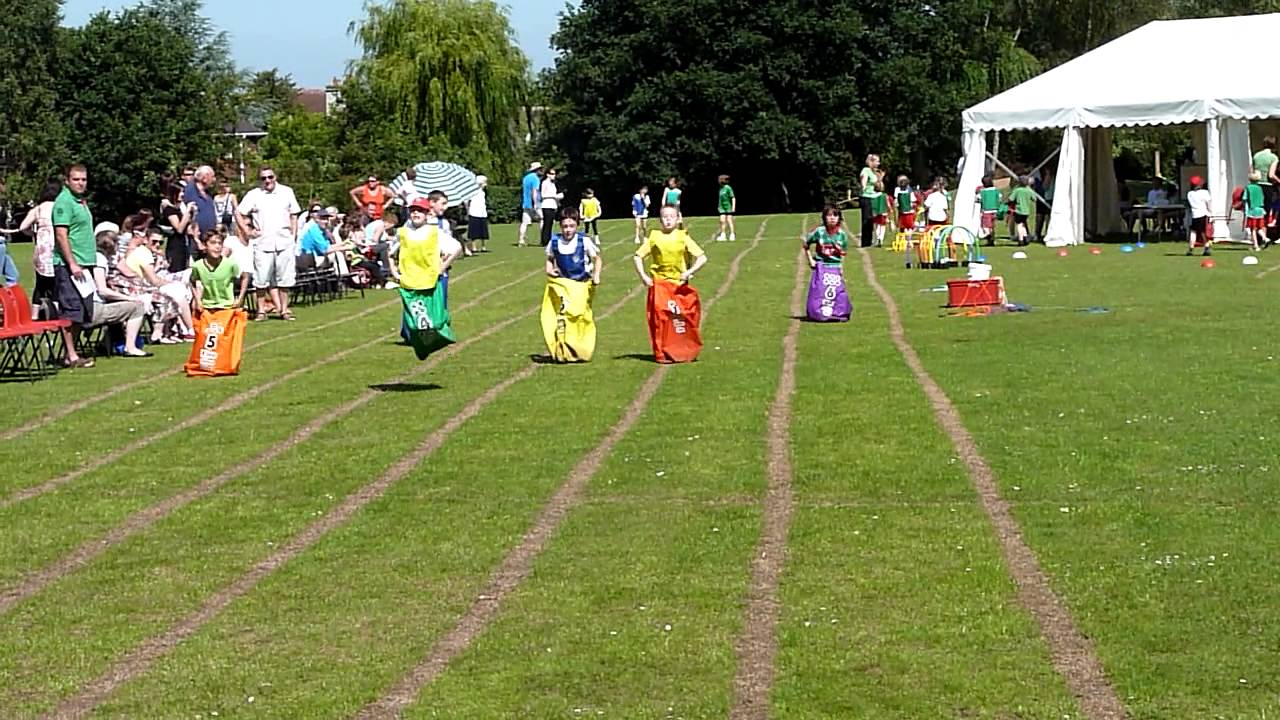This outdoor photo captures a lively scene of a sack race competition involving five children, each wearing a colorful gunny sack (orange, green, yellow, red, and purple) with numbers written on them. The race is taking place on a grassy field lined with trees and large tents, indicative of a picnic or organized event. The children, energetically hopping in their lanes, are surrounded by an audience of parents, relatives, and friends seated on the sidelines, cheering them on. In the background, more adults and kids can be seen along with toys, adding to the festive atmosphere. The positioning in the image shows the racers in the center, with grassy areas below and to the right, a tent pavilion in the top right corner, and a backdrop of trees stretching from the top center to the left.